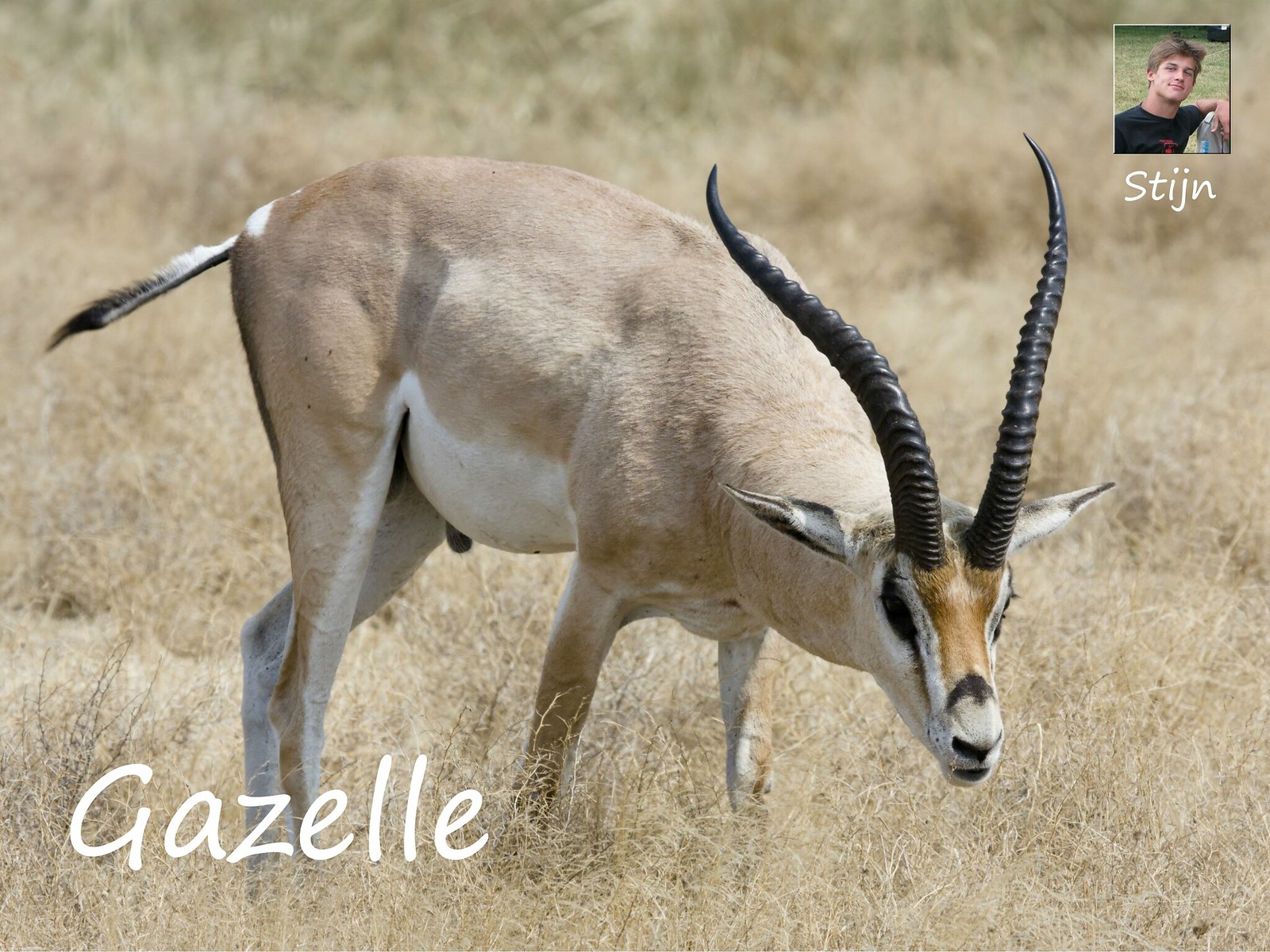The photograph captures a graceful gazelle poised in a flat field of tall, dried yellow grass, resembling wheat. The gazelle's deer-like body features a tan back, transitioning to a white stomach and lower legs. Its face is adorned in a rich golden hue, accented by white markings and a distinct black spot on its nose. Long, spiraling horns, dark and coming to sharp points, extend from its head, while its ears extend outwards. Although the hooves are obscured by the surrounding grass, the gazelle's short tail, marked with black and white, is visible. In the bottom left corner of the image, the word "gazelle" is prominently displayed in white font. Meanwhile, the top right corner features a photograph of a man with the name "Stigeon" written beneath it, suggesting he may be the photographer or the image's creator.